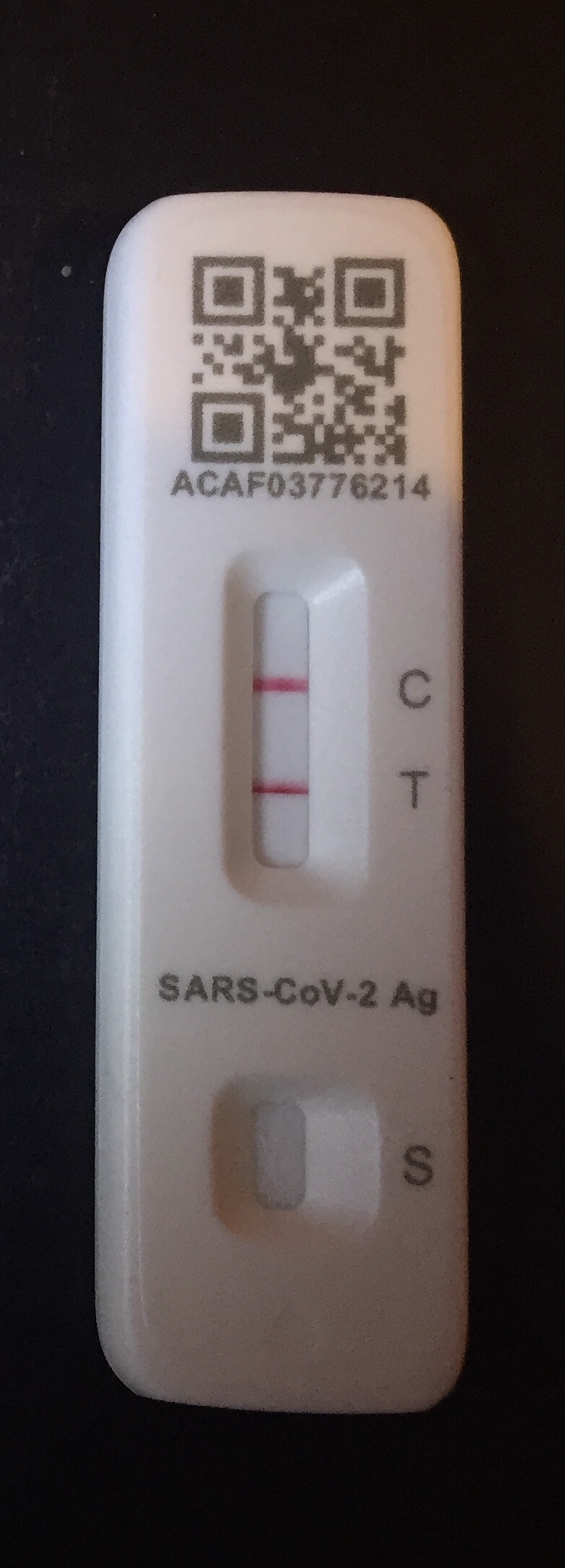The image features a SARS-CoV-2 antigen (AG) rapid test device, designed to detect active COVID-19 infection. The test device, made from white plastic material, prominently displays a QR code at the top, followed by a unique alphanumeric code: ACAF03776214. Directly below the QR code, the test panel shows results, indicated by two red lines beside the letters 'C' (control) and 'T' (test), confirming a positive result for the virus. The inscription "SARS-CoV-2 AG" is located beneath the result panel, and further below is a small well, marked with the letter 'S' for 'sample,' where the test sample is to be deposited. The stark black background isolates and highlights the test device, emphasizing the critical information presented.